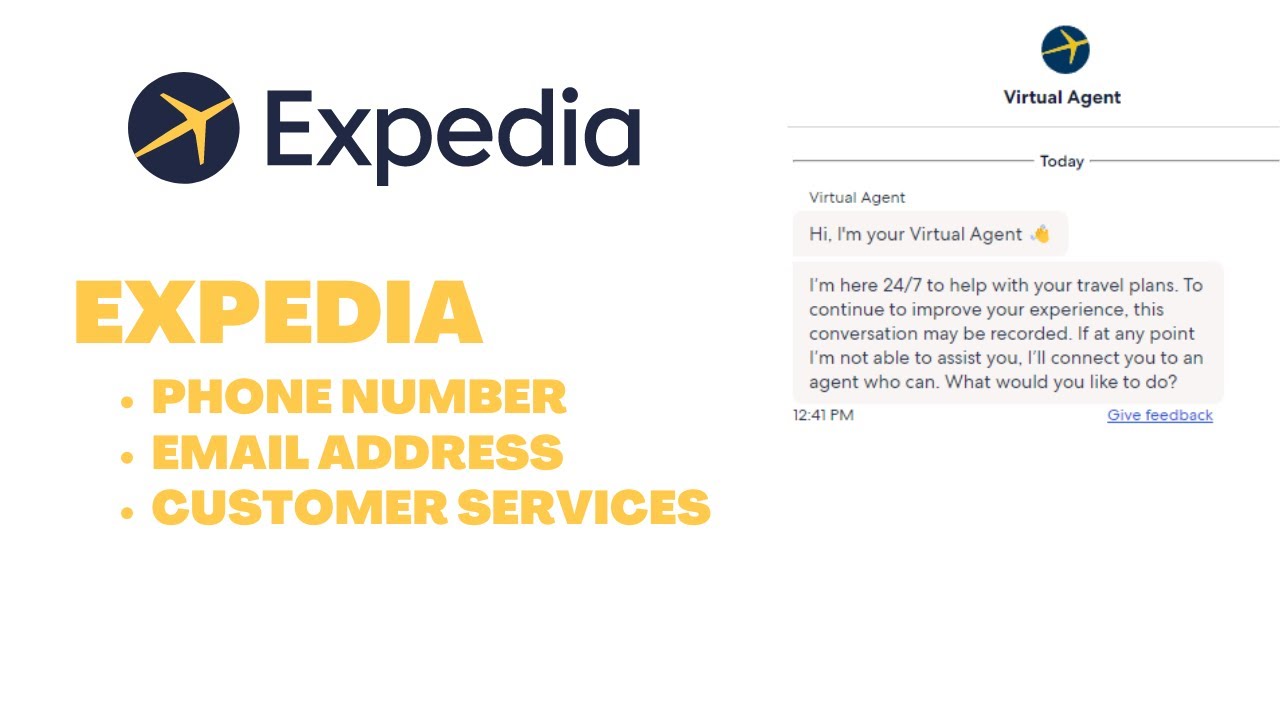The image, sourced from Expedia's website, features a pristine white background divided into two distinct halves. The left half is unique and contains several prominent elements. Near the top left corner, there is a large blue circle. Just below the circle, extending toward the upper right, is an outline of an airplane rendered in a goldish hue, with its wings angled upward to the left and downward to the right. Adjacent to the airplane outline is bold black text that reads "Expedia," followed by a repetition of "Expedia" in gold, all in capitalized bold letters.

Below this gold "Expedia" title are several categories, each separated by a dot:
- All caps, bolded "PHONE NUMBER"
- Dot
- All caps, bolded "EMAIL ADDRESS"
- Dot
- All caps, bolded "CUSTOMER SERVICE"

The right half of the image is centered around marketing and assistance features. Prominently, in the middle section, the circle emblem from the left reappears. Directly beneath it, the words "Virtual Agent" are displayed in black text. This is followed by a thin blue line that crosses from the center to the right, interrupted by the word "Today" in black, before continuing towards the right edge.

Below this, against a white background aligned to the left, a conversation is illustrated inside a light blue talk rectangle with dark blue text that reads, "Hi. I’m your virtual agent," concluded with an indiscernible emoji. This is followed by another light blue rectangle containing several lines of conversation aimed at assisting with travel plans.

Toward the bottom left, in smaller dark blue text, the timestamp "12:41 p.m." is provided. On the right side, the word "Give feedback" appears in blue and underlined, indicating it is a clickable link.